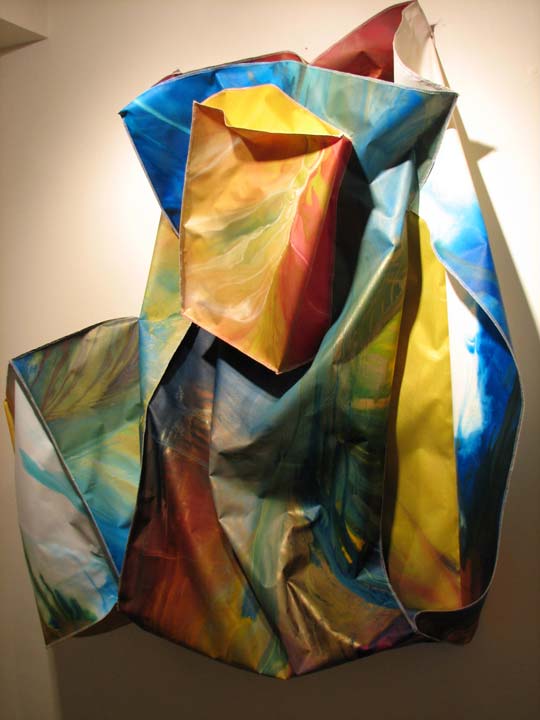The image showcases a highly detailed and vibrant painting of a crinkled, folded bag hanging on a nail against a tan-colored wall, possibly within a museum gallery setting. The bag displays an array of bright, vivid primary colors, including blue, red, yellow, and green, arranged in an intricate, almost rainbow-like design. These colors are distributed across multiple smaller and larger sections of the bag, creating a unique and eye-catching pattern. The largest section features a mix of colors: red in the bottom left corner, blue on the right, with a golden bottom and light blue top. A smaller, orange-yellow rectangular bag is positioned near the top, with red sides and a yellow interior. Another bag behind it contributes additional colors: white on the outside, with light brown, blue, and yellow on the inside. The interplay of these colors enhances the visual interest and emphasizes the texture of the bag, which appears almost three-dimensional due to its shadow and the light source above.